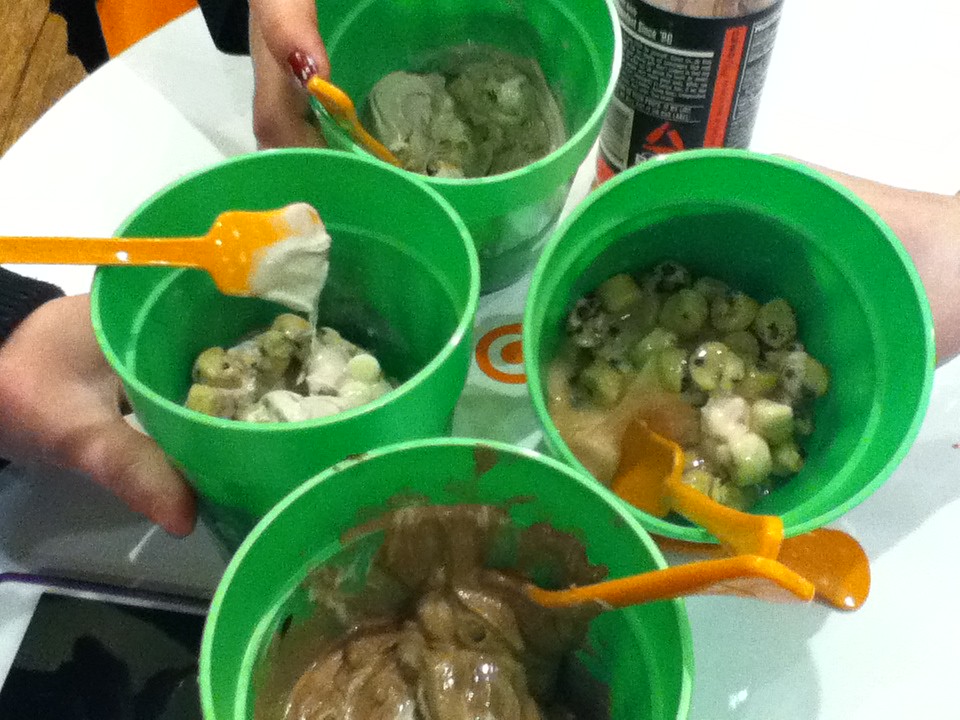This color photo, taken from an overhead perspective, captures four green plastic cups filled with various types of ice cream or frozen yogurt, each with orange shovel-shaped spoons. The cups are arranged closely together on a white table, suggesting a sense of camaraderie among the friends. The ice cream flavors appear diverse, with the front cup containing a brown, pudding-like substance, possibly chocolate, with an orange spoon inside. The cup to the left features white ice cream with an array of chopped toppings, mirrored by another cup across, loaded with even more toppings. At the top of the image, a hand with red nail polish holds a cup containing a gray-green ice cream, adding an interesting color contrast. Scattered on the table are phones and what seems to be a drink with a vague Target logo, implying the group may have visited the store. The scene evokes a casual and friendly gathering, capturing a shared moment of indulgence.